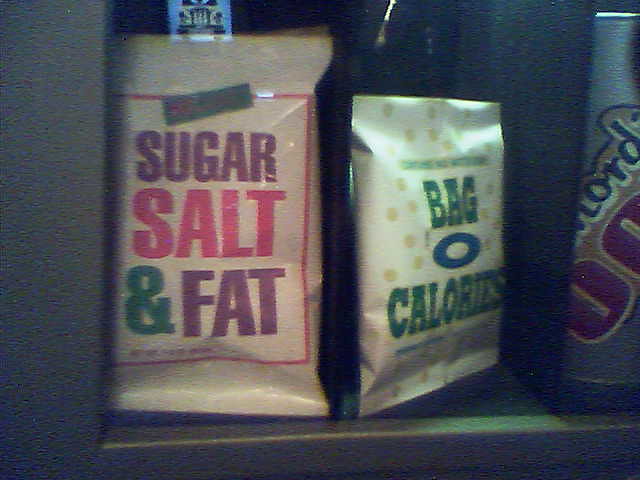This photograph captures the inside of a kitchen cabinet, humorously staged to critique common snack choices. The shelf is lined with various satirical snack products. On the left, there's a tan-colored bag labeled "Sugar, Salt, and Fat" in purple, pink, and green writing, highlighting unhealthy ingredients often hidden in snacks. Prominently positioned in the center, a white bag labeled "Calories" features green text and a blue circle, further emphasizing the caloric content of such foods. In the background, multiple other packages reinforce the theme with their unrealistic and comedic labels. To the right, a bottle possibly containing soda adds to the array of unhealthy choices typically hidden in kitchen cabinets. This witty setup sends a clear message about the hidden nutritional pitfalls of common snacking options.